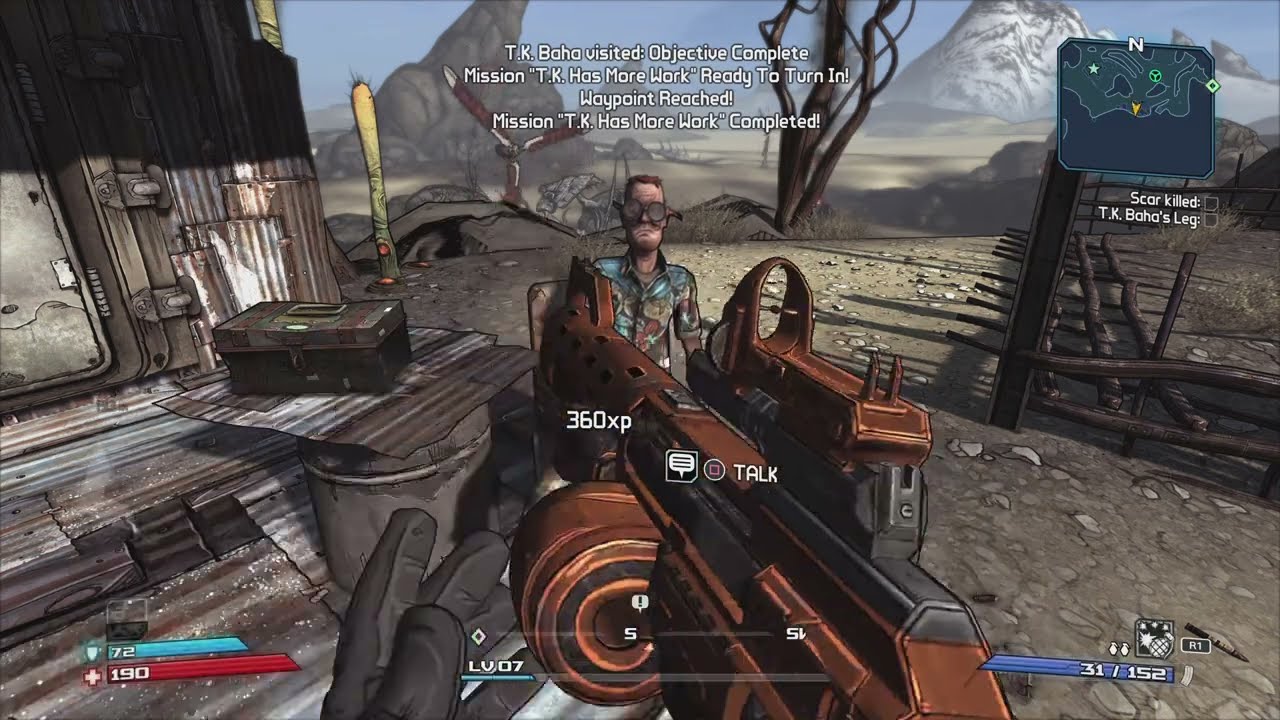In this detailed screenshot from the video game "Borderlands," the scene presents a vivid post-apocalyptic, Mad Max-inspired setting. The foreground features a first-person view of an orange and black rifle with a large drum magazine and a sight circled in bronze, held by a character wearing black leather gloves. The gun displays a capacity of 152 bullets. Text overlays at the top of the screen read “TK Baja visited. Objective complete. Mission TK has more work ready to turn in. Waypoint reached. Mission TK has more work completed,” indicating completed objectives.

The central figure in the frame is a white male character with short red hair, wearing large round goggles and a blue tropical floral Hawaiian shirt. He sits in a makeshift chair beside a shack constructed from corrugated steel and other scavenged materials. The environment consists of gray stone and gravel, typical of a desert wasteland.

Additional HUD elements include a health bar and armor indicator in the bottom left, a grenade icon in the bottom right, a map with direction icons in the top right, and the player’s level displayed in the center. The colors in the image encompass a range of brown, gray, red, light blue, dark blue, tan, black, and white, all contributing to the game’s unique and immersive aesthetic.